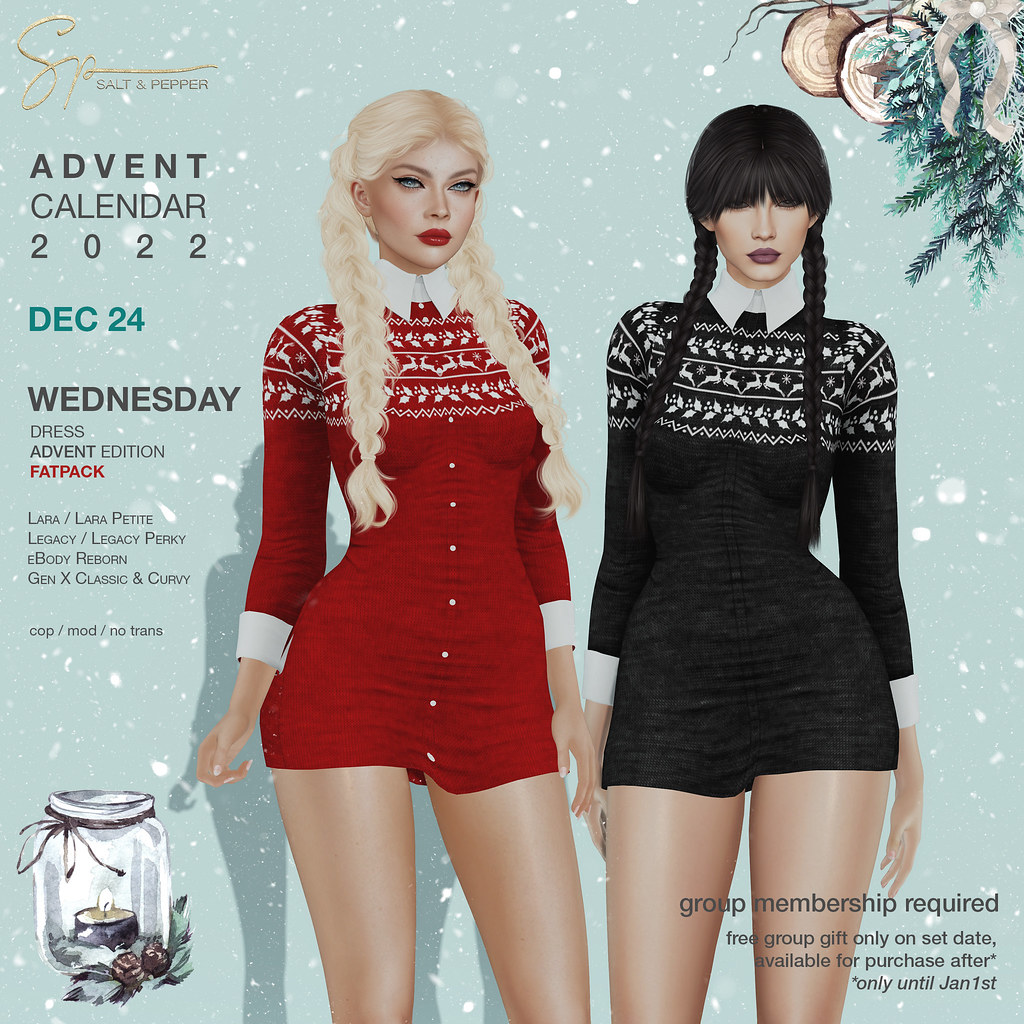The image is an advertisement for the SP Salt and Pepper Advent Calendar 2022, featuring a promotional group membership requirement. In the center, two models stand facing the camera, each with hair braided into long pigtails. The blonde model, styled with no bangs, wears a short, red Santa-themed dress with a white button-down shirt underneath, complemented by heavy makeup and red lips. The black-haired model, adorned with bangs, dons the same outfit in black with a pink lip shade and similarly heavy makeup. Both dresses are long-sleeved and cut off at the crotch, leaving their legs bare. Additional festive elements like Christmas decorations, holly with logs and ribbons, and a candle illustration with small pine cones embellish the advertisement. The top left displays the store's name, "Salt and Pepper," while the text on the ad reads, "Advent Calendar 2022," "Group membership required, free group gift only on set date, available for purchase after only until January 1st." The vivid colors include red, black, white, light blue, gold, turquoise, gray, and silver, giving the ad a holiday and fashion-centric appeal.